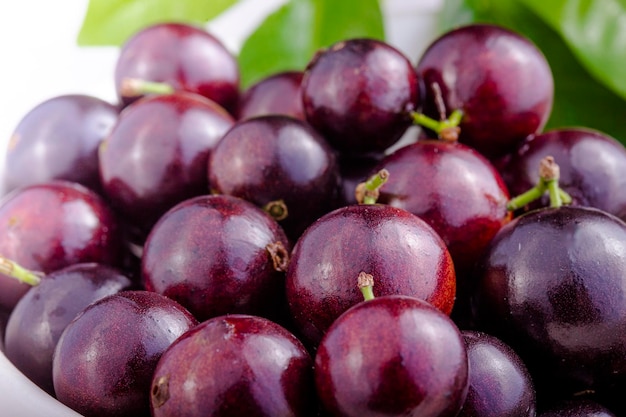The close-up photograph captures a bunch of ripe, glossy grapes, predominantly dark purple in color with varying shades of richer reds in the middle. They are round in shape and exhibit a noticeable shine due to the light source coming from the upper right. The grapes are attached to thin green stems that bring some of them together. In the foreground, on the lower left, a white curve resembling the lip of a plastic bowl can be seen, suggesting the grapes may be in a container. The background features three distinctly colored leaves: a lighter lime green leaf on the left, a richly colored one in the middle at the top, and a darker green leaf on the upper right. The scene is closely focused on the grapes, showing their detailed texture and ripe appearance, giving them a very appetizing look.